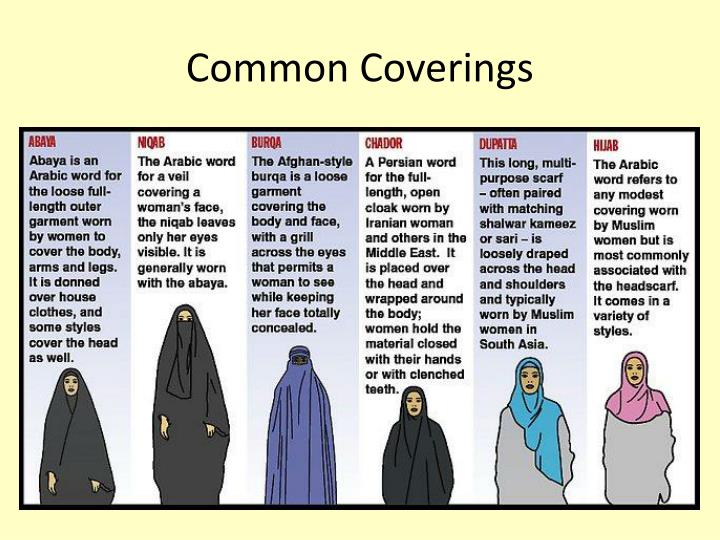This vibrant infographic, set against a yellow backdrop, details the diverse coverings worn by women in the Middle East and South Asia. The title "Common Coverings" is highlighted in black text at the top center. From left to right, six sections depict different garments with corresponding descriptions written in black and red text.

1. **Abaya**: Illustrating an Arabic term for a loose, full-length outer garment, typically black, that covers the body, arms, and legs. It is worn over everyday clothes, with some styles extending to cover the head as well. 

2. **Niqab**: Shown as a veil covering a woman’s face, leaving only the eyes visible, and is commonly paired with an abaya. This traditional Arabic garment is also predominantly black.

3. **Burqa**: Represented in a bluish-purple hue, this Afghan-style garment entirely conceals the body and face, featuring a grill across the eyes that allows the woman to see while maintaining full coverage.

4. **Chador**: This section, illustrated in black, describes the Persian term for a full-length open cloak, often worn by Iranian women. It is draped over the head and wrapped around the body, with the material held close by hands or clenched teeth.

5. **Dupatta**: Depicted with a light blue head covering, this long, multi-purpose scarf is often matched with traditional outfits like shalwar kameez or sari. It is loosely draped across the head and shoulders, mainly worn by Muslim women in South Asia.

6. **Hijab**: With a light pink head covering, this term refers to any modest attire worn by Muslim women but is most commonly associated with the headscarf. It presents in various styles and is simply draped to cover the hair and neck.

Each section features a cartoonish illustration of a woman wearing the respective covering, providing a clear visual reference to accompany the detailed descriptions.